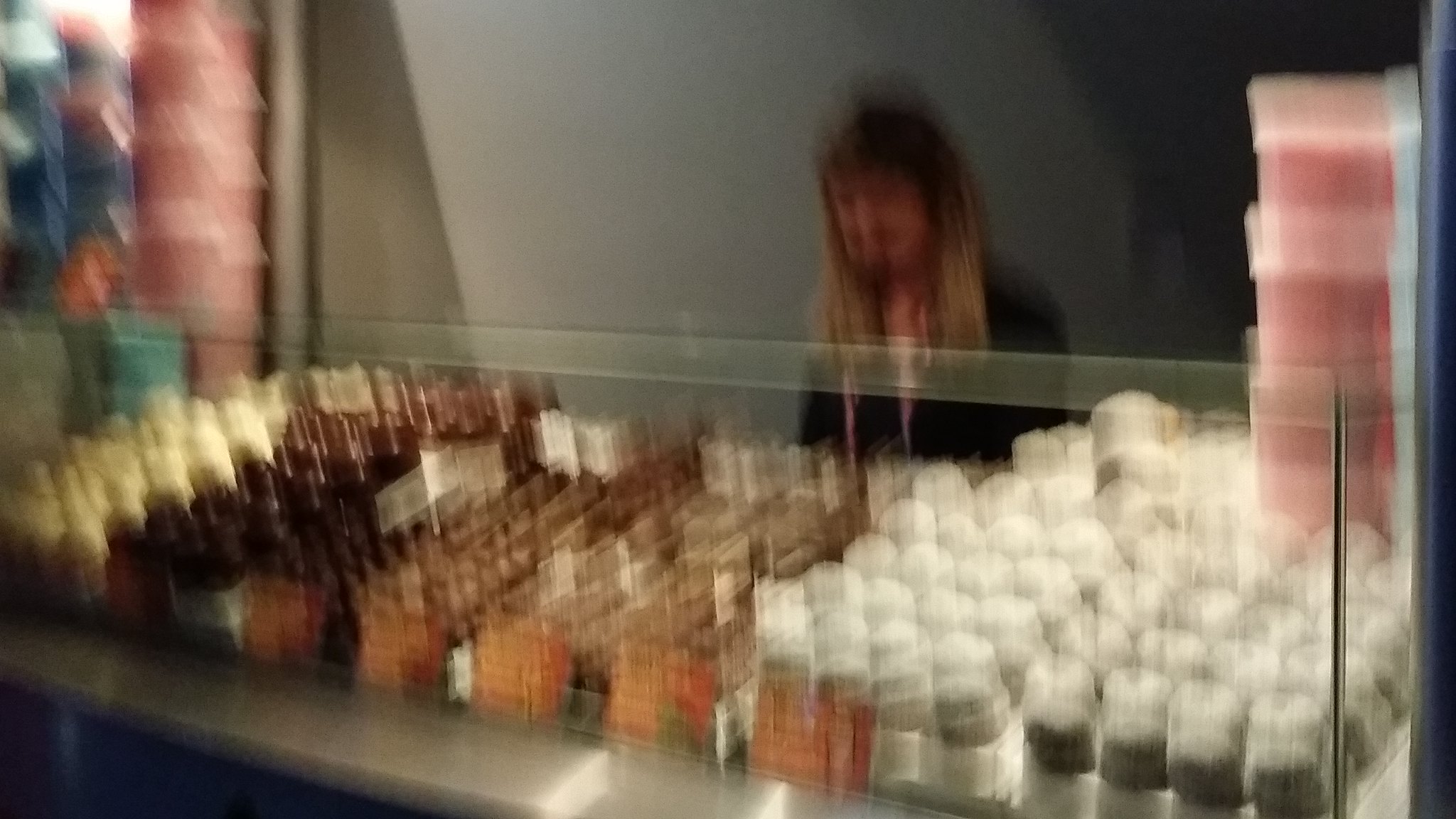This photograph depicts a woman standing behind what appears to be a counter in a bakery or candy store. The image quality is very poor, making details challenging to discern. The woman, who seems to be Caucasian, has a mix of brown and blonde hair and is dressed in a dark sweater layered over a cardigan. She appears to be situated against a gray wall backdrop. To her left and right, there are stacks of what look like pink cotton candy. On the right side of the image, there are items that resemble chocolate-covered marshmallows and possibly white chocolate or white cupcakes, although the blurriness obscures these details. The scene has a chaotic, fuzzy quality, leaving much to the observer's imagination.